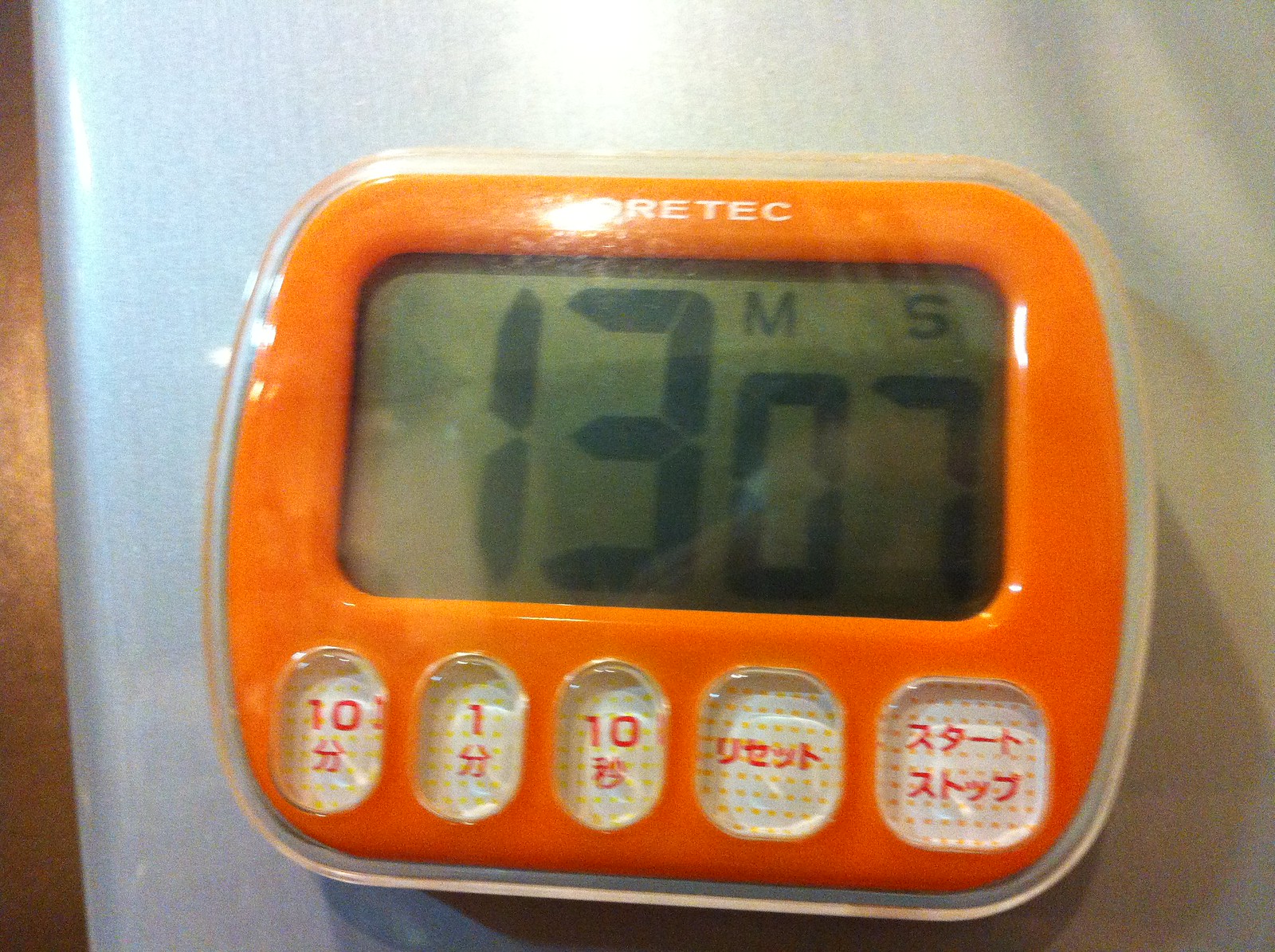The photograph depicts a small, orange-colored digital timer or alarm clock with a notably clear border around its square, rounded-edged frame. The device's rectangular LCD screen displays "MS" in the top right corner and the time "13:07." Below the screen, there are five buttons with numbers (10, 1, 10, 1, and 10) and Chinese characters. The first three buttons read 10, 1, and 10 respectively, while the fourth appears to indicate "test," and the fifth possibly functions as a start-stop button. The device sits on a white surface, which could be a countertop or shelf, with a brown background behind it. There is a noticeable glare on the screen and top part, partially obscuring the brand name, which appears to start with "RETEC." Additionally, there is a white wall behind the device with a vertical brass trim on the left side, suggesting a room or wall divider.